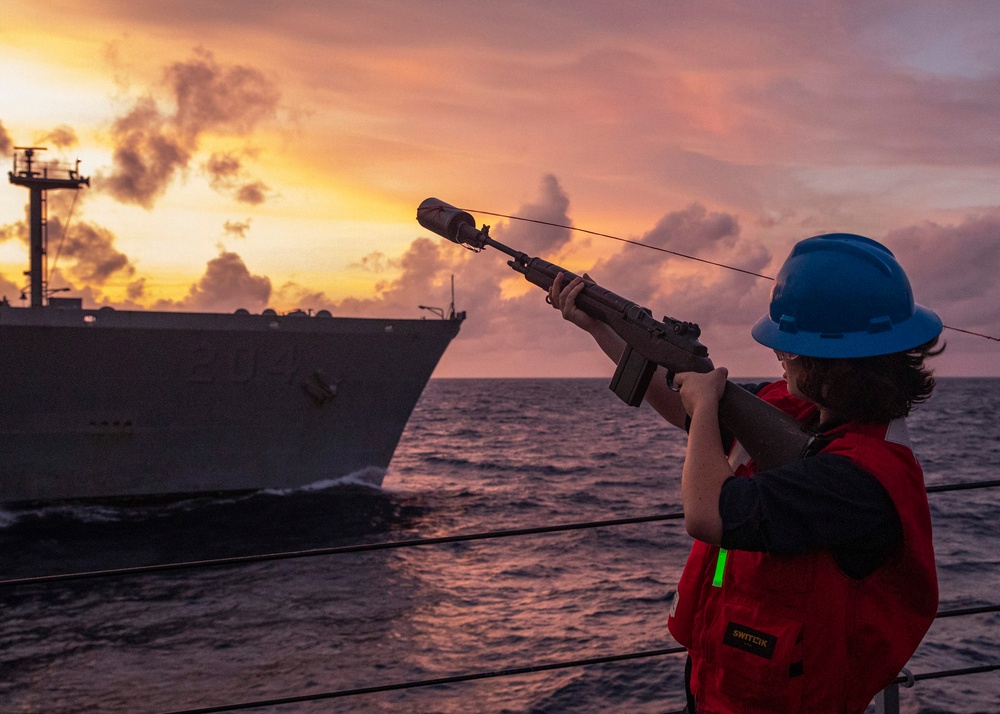The image captures a dynamic maritime scene at sunset, dominated by a striking gray ship marked with the number 204. It's silhouetted against a vibrant sky awash with hues of bright yellow, orange, pale pinks, and light blues, with clouds hovering on the horizon. In the foreground, an individual of ambiguous gender, possibly female, is standing on the deck of another vessel amidst the surrounding ocean waters. This person is adorned in an orange life vest, a blue hard hat, and a black shirt with sleeves that reach their elbows. Their medium-length brown hair flows to their shoulders. They hold a peculiar rifle-like apparatus, the tip of which features a large cork connected to a cable, suggesting it's used for launching a tow line. This scene, illuminated by the fading light of a setting sun, hints at a potentially critical operation between the two ships, underscored by the beautiful yet serene maritime backdrop.